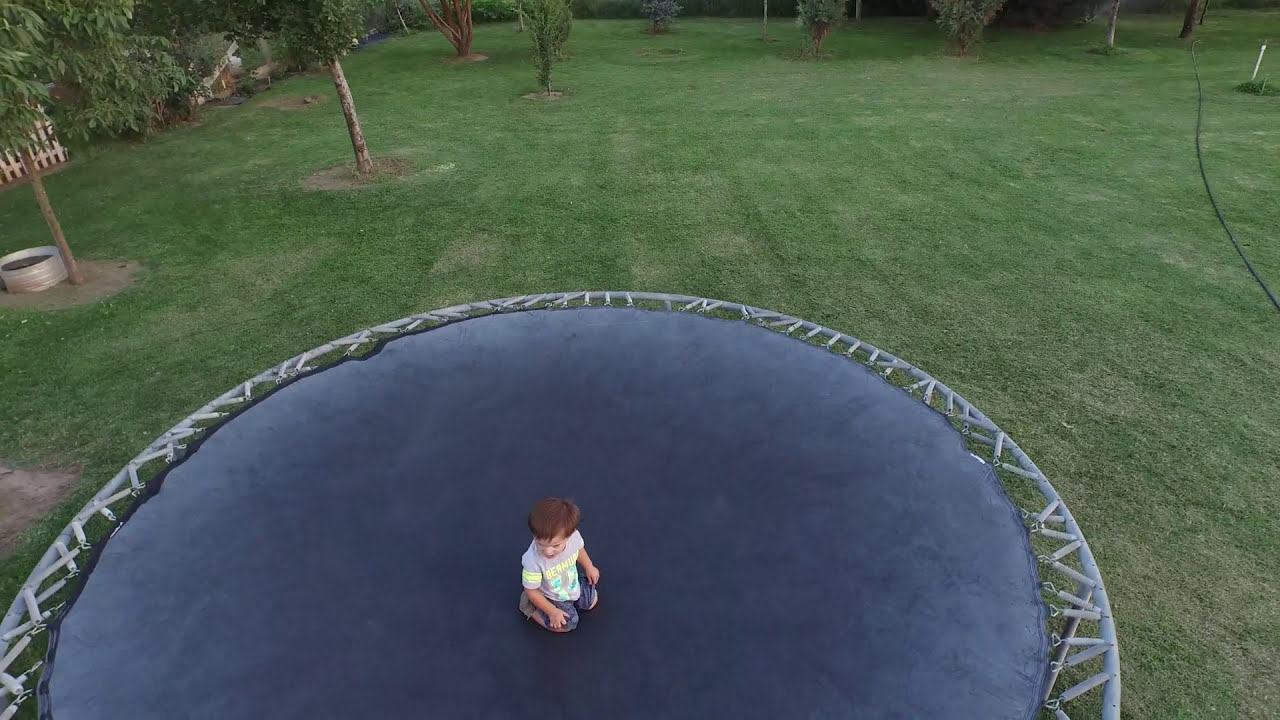In a spacious and well-manicured backyard, a young boy, likely around four years old, is pictured on a large, blue trampoline. He is dressed in a lavender shirt with a yellow stripe and shorts, and he is sitting on his knees at the center of the trampoline. The trampoline lacks modern safety features, such as a net or enclosure. The yard, which has neatly cut green grass and several small trees, provides a serene backdrop. On the upper right side of the image, a dark-colored hose and an indistinct object are visible. Additionally, there is an aluminum item, possibly a round container with dirt, near one of the trees. The background also features a white picket fence and some larger trees marking the yard's boundary. The boy, who appears to have red hair, looks to his right, and no other people are present in the scene. The main colors in the image are green, brown, white, and blue.